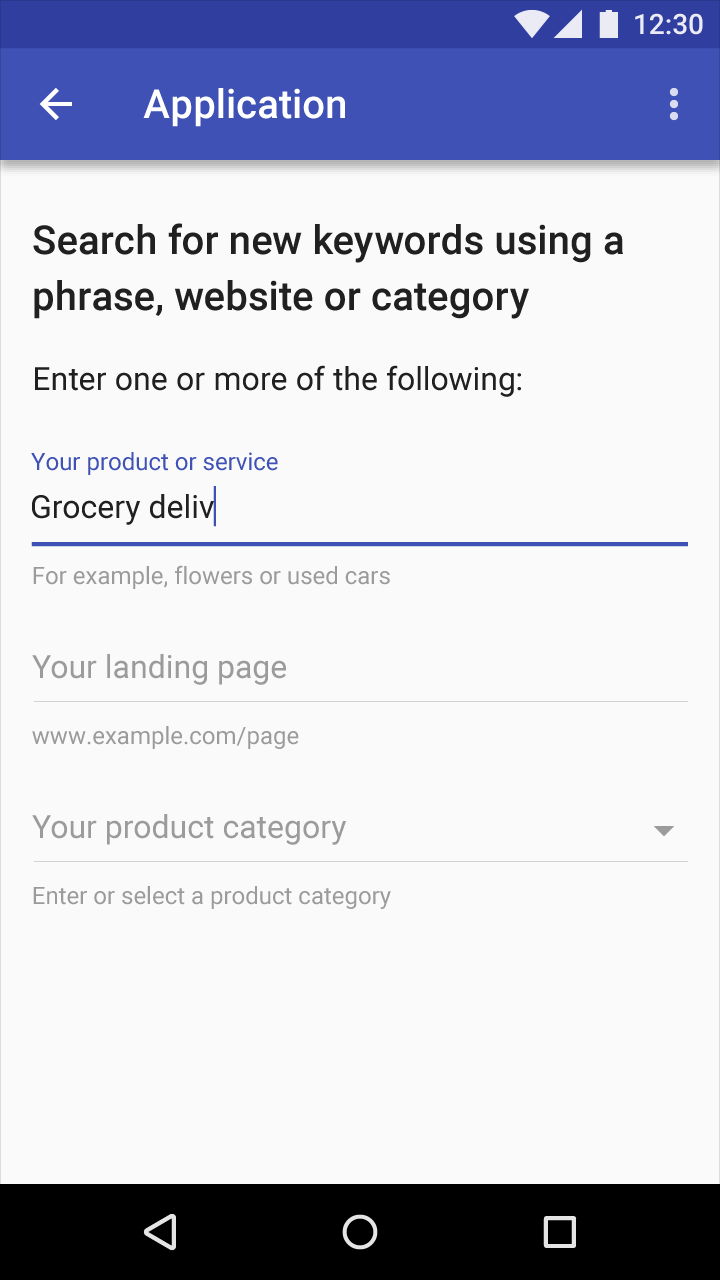The image depicts a mobile phone interface that is likely running on an Android or Google-based system, characterized by the common design elements of these platforms. At the top left of the screen, there's an arrow allowing the user to navigate back, and on the right, there's a kebab menu (three vertical dots) indicating additional options.

The main title of the page reads "Search for new keywords using a phrase, website, or category." Beneath this, the subtitle provides further instructions: "Enter one or more of the following." The form includes fields to input details about a product or service, with examples such as "flowers" or "used cars." Another section prompts the user to enter a "landing page," providing an example format like "www.example.com/page." The final dropdown allows the selection of a product category, guiding the user to "enter" and "select a product category."

The screen is evidently designed for users to input information about a business, product, or service, although the specific application or purpose is not clear from the context provided. On the top right corner of the interface, the time is displayed as 12:30 (unspecified whether AM or PM), along with icons indicating the device’s Wi-Fi connectivity, battery level, and a triangular symbol pointing left, the latter of which is not immediately identifiable.